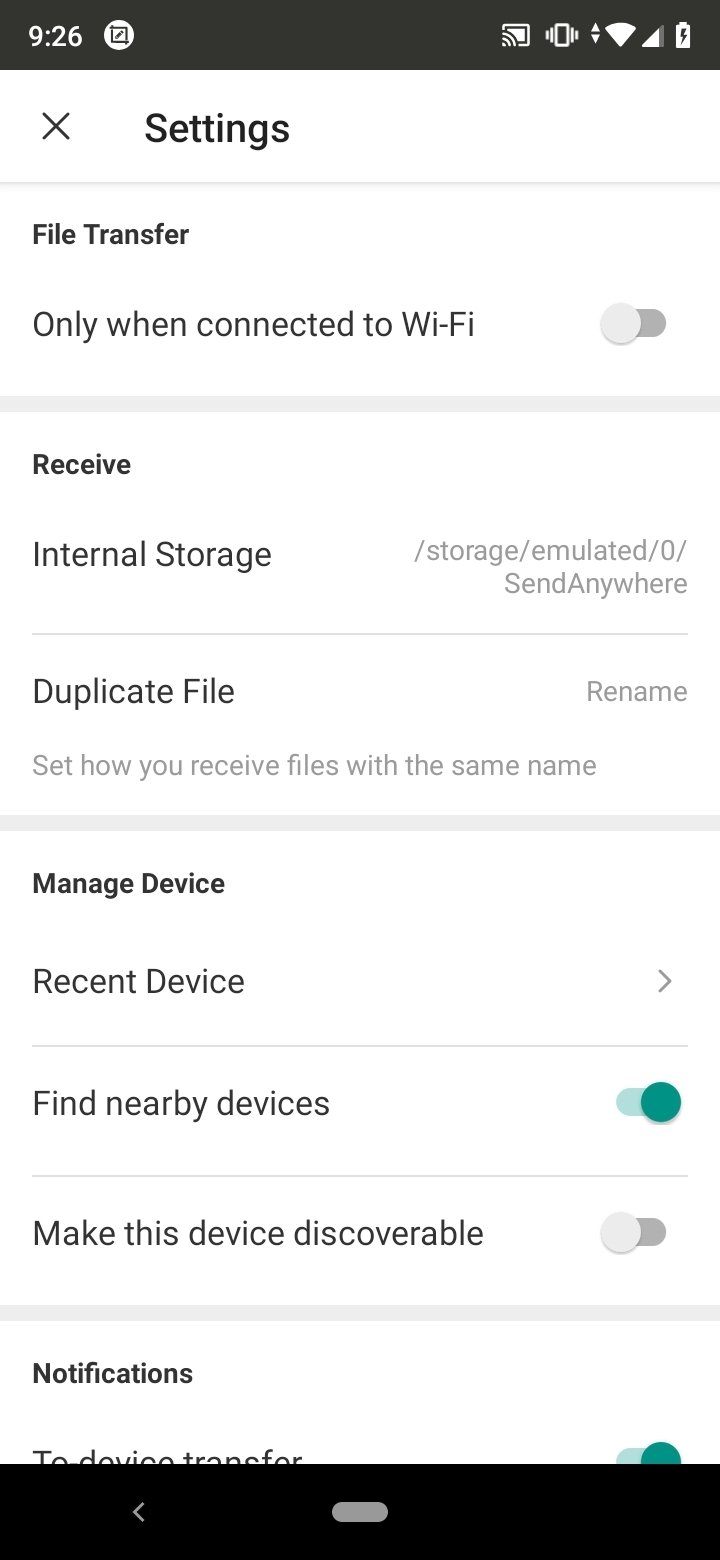A smartphone screenshot captured at 9:26 (AM or PM unknown) shows the device's settings interface displayed on a black banner. The battery indicator is critically low, signaling the need for a recharge. The current settings page features options related to file transfer. The first visible option, "File Transfer," allows file transfers only when connected to Wi-Fi, though this setting is turned off. The "Receive" option is set to internal storage, providing various file management choices such as "Duplicate file" with the option to rename duplicates, and manage storage.

Key interface sections are marked in a darker font, including "Manage Device," "Receive," and "File Transfer." Under "Manage Device," there is an option for "Recent Device" which allows users to switch between recently connected devices. The "Find Nearby Devices" function is enabled, making the device capable of interfacing with nearby devices. However, "Make this device discoverable" is turned off, preventing it from being found by other devices. The lower part of the screen hints at notifications related to file transfers, though the text is partially obscured. A black bar is present at the bottom of the screen.